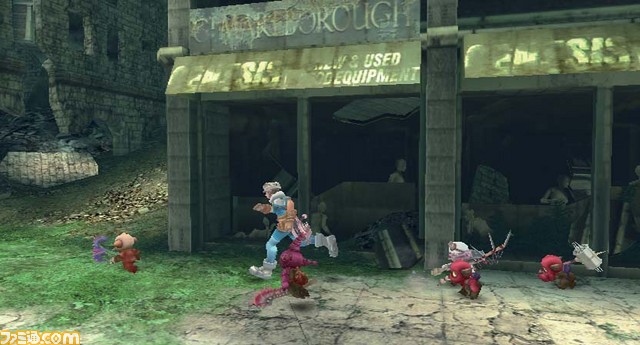The image is a screenshot from the Nintendo Wii game "Earthseeker." It depicts an outdoor scene set in what appears to be an abandoned ruins area. On the left side, there's a broken-down wall of a castle-like structure, made of gray stones and featuring large windows. Below this structure is a grassy area interspersed with dirt, gradually ascending a slope. In the center of the image stands a building constructed of cinder blocks, with four large windows prominently displayed.

The foreground showcases several small creatures, resembling gnomes or robots, in various colors such as pink, tan, burgundy, and purple. Some of these creatures are holding weapons. Amidst these characters is a larger figure dressed in blue and brown attire, with white boots, seemingly the main character of the game, running through the scene. The right bottom corner of the image reveals light tan and black-colored stone or concrete, adding to the detailed, pre-rendered look of the environment.